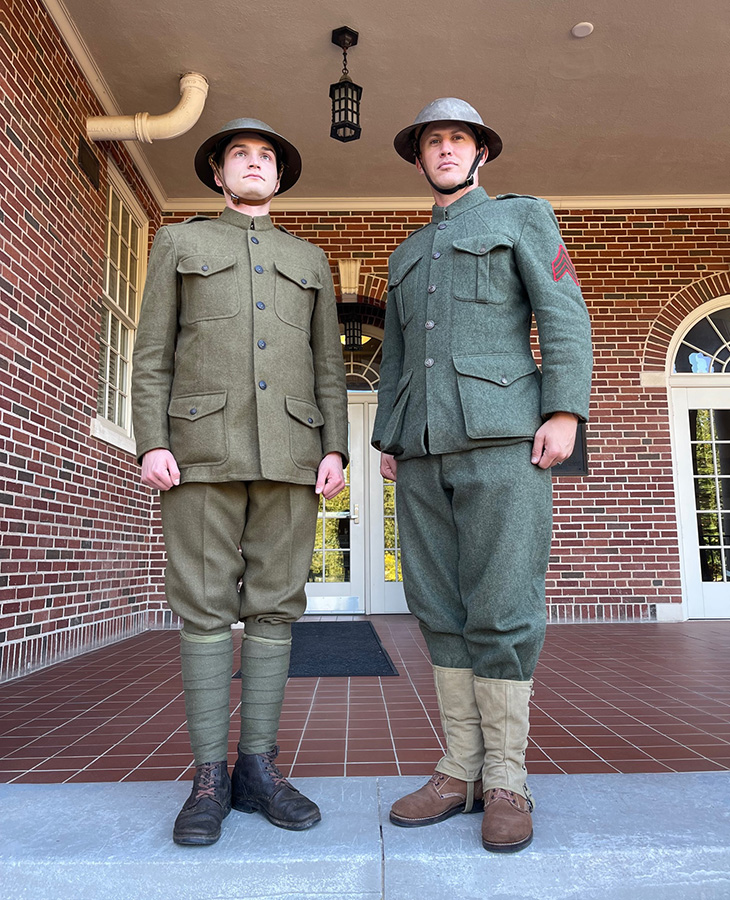This image depicts two soldiers standing on a cement porch in front of a large red brick building with white-framed doors and windows. Both are dressed in old-fashioned military uniforms and helmets, appearing somewhat like mannequins or sculptures owing to their static poses and facial expressions. The soldier on the left wears an olive-green, buttoned-up coat with matching pants, black boots, and green wraps above the boots. The soldier on the right wears a light blue military jacket and pants, tan wraps around his brown boots, and bears a distinctive red arrow insignia on his sleeve. They stand side by side, gazing straight ahead, somewhat away from the camera. Behind them are white double doors leading into the building, highlighted by a visible white ceiling. The scene is staged on a dark red paver area, suggesting a formal or historical setting, possibly a museum or a commemorative site.